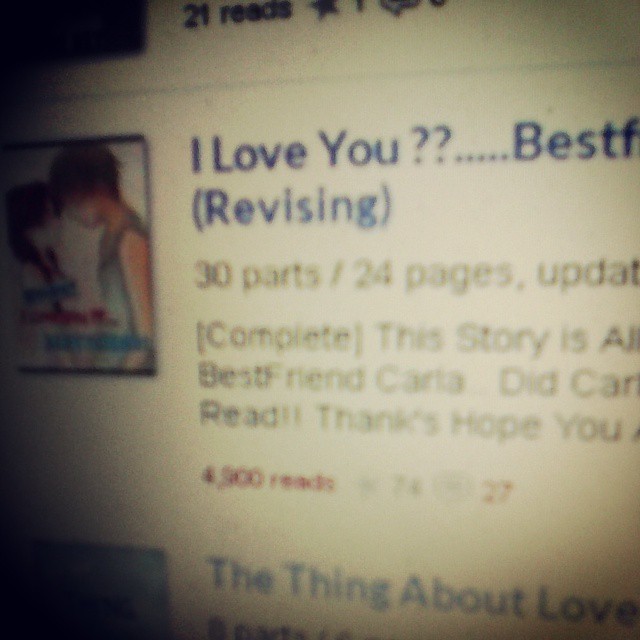The image appears to be a screenshot from a computer or mobile device, primarily featuring a web page with a white background. On the left side of the screen, there is an image showcasing anime characters, a boy and a girl. On the right side, a prominent blue heading reads “I love you...” followed by an ellipsis. Below this, there is text indicating the content is titled “Best Web (Revising).” Further details below the heading specify "30 parts / 24 pages," and it is marked as completed. The description notes that the story involves a best friend named Carla and adds a thank you message with “hope” included. The page shows it has received 49,000 reads. Additional smaller articles are visible at the top and bottom of the screen; the top article has 21 reads and the bottom article is titled “The Thing About Love.” The overall image quality is blurry, making it difficult to discern finer details, but it indicates a focus on digital content related to anime and story publications.